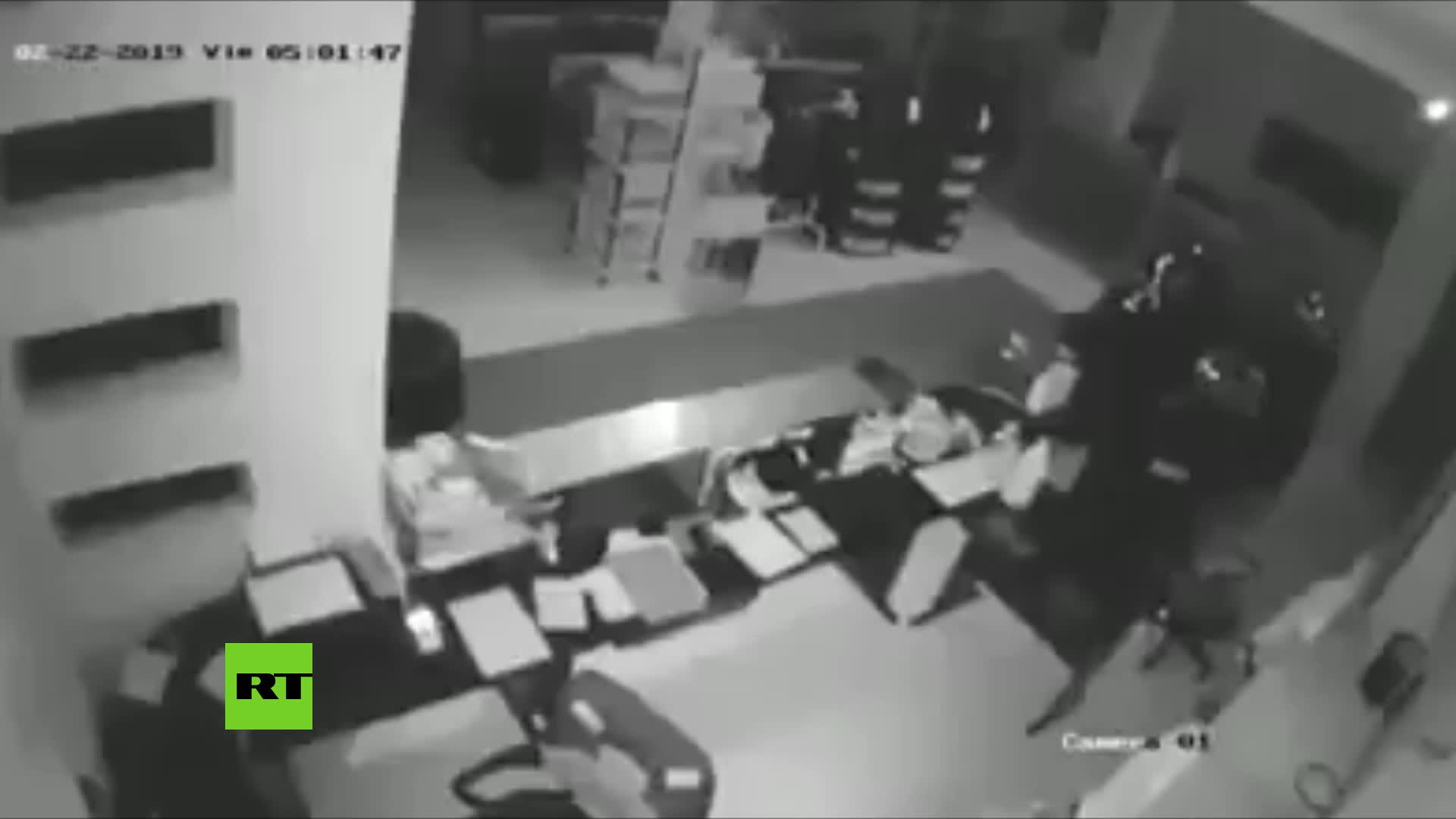The black-and-white screen grab from a surveillance camera, labeled "Camera 01" in the bottom right corner, shows an office or business setting illuminated by dim lighting. Captured on 02-22-2019 at 05:01:47, as indicated by the timestamp at the top, the image presents a somewhat foggy and indistinct view. The lower left corner features a green rectangle with the black text "RT," marking it as displayed on Russia Today. Central to the image is a long desk cluttered with numerous papers, suggesting an active workspace. To the right, large, dark, and indistinct shapes can be spotted, possibly representing rolling carts with shelves and other equipment. A white pillar with three dark openings stands to the left, hinting at a structural element of the room. The tile floor includes a noticeable line pattern, while the overall clarity of objects within the scene remains low, adding to the mysterious and somewhat cluttered atmosphere.